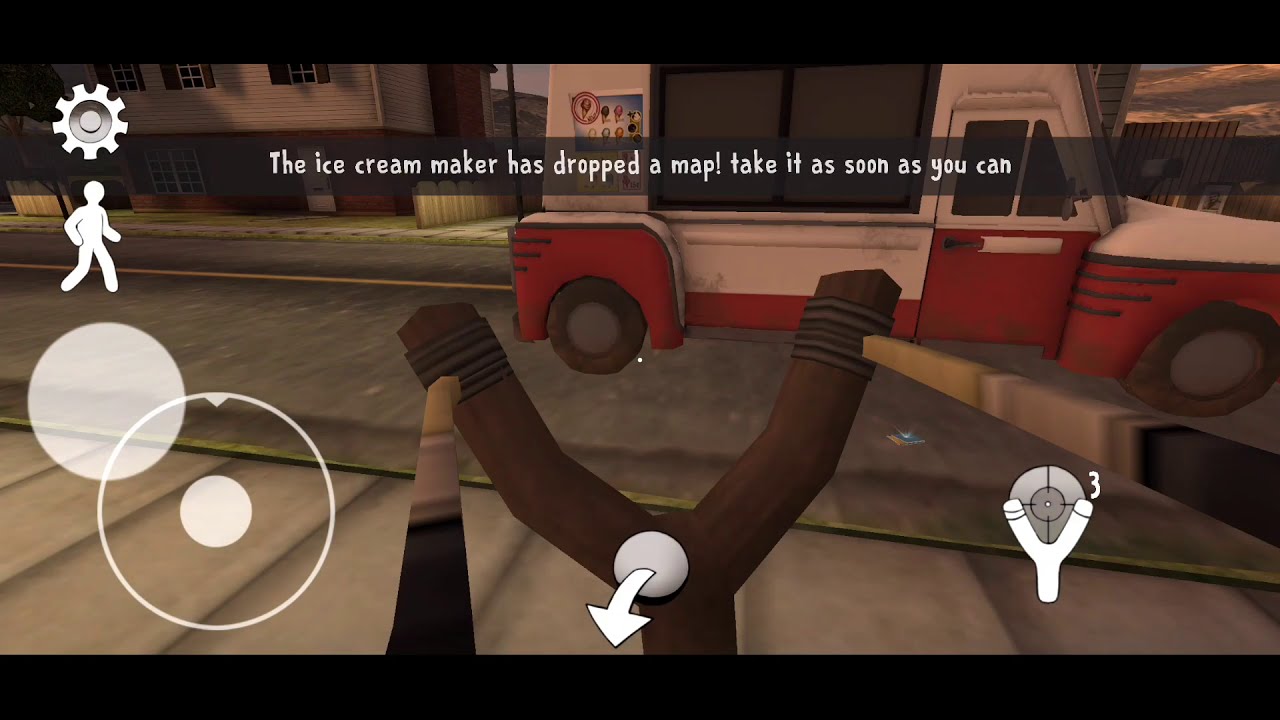This detailed screenshot captures a nostalgic, blocky-style 3D video game featuring a first-person perspective of a player aiming a wooden slingshot. The scene is set on a street with a red and white ice cream truck, adorned with various stickers depicting ice creams, positioned in front of a backdrop of houses. The slingshot, prominently held by the player, occupies the lower part of the image, its elastic bands drawn back and ready to shoot. In the upper left corner, various on-screen controls and icons indicate player settings: a gear symbol, a human figure, and two interspersed circles. The lower right corner displays an ammo counter alongside a slingshot icon with the number three, signifying the remaining shots. At the top of the screen, a message in white text reads, "The ice cream maker has dropped a map. Take it as soon as you can." This further sets the objective of the scene, urging the player to act swiftly amidst the vintage, Nintendo 64 reminiscent graphics, which lend the game a charming, cartoon-like quality despite their deliberately blocky appearance.